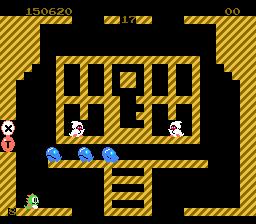This image appears to be a screenshot from a video game reminiscent of Pac-Man. The background is primarily black with accents of yellow. At the top left corner, the score prominently displays "150,620," while the top right corner shows two zeros ("00"). Centrally located in the middle of the image is the number "17." On the left side, also near the middle, are the letters "X" and "T." The scene depicts a maze populated by various cartoonish characters resembling an off-brand version of Pac-Man. Two ghost-like white characters navigate the maze, seemingly in pursuit. Beneath them are smaller blue characters whose roles are unclear. At the bottom of the image, a green character stands alongside the numeral "8," further emphasizing that this game is a variant of the classic Pac-Man format.